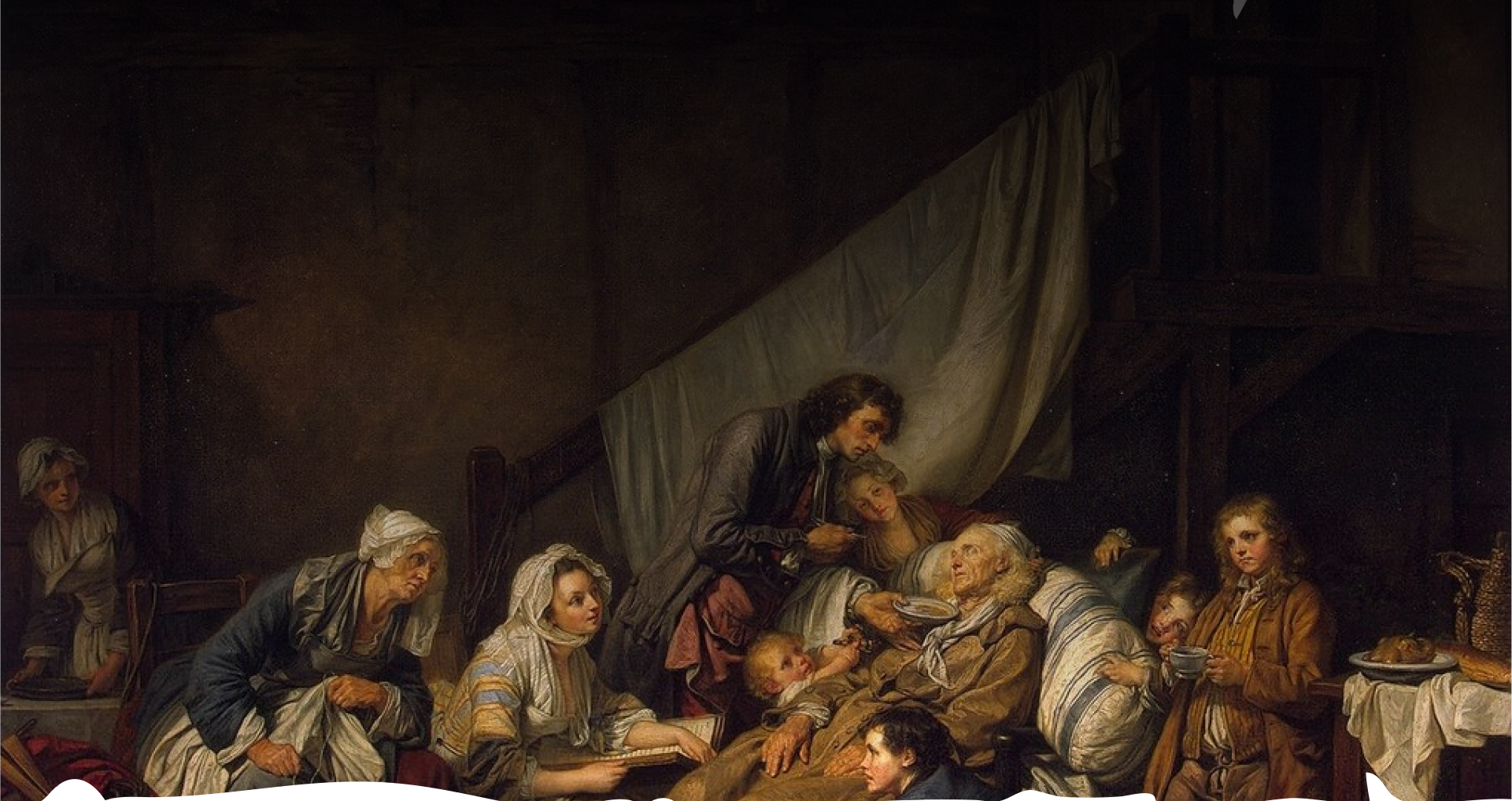The painting depicts a group of people in a dimly lit room characterized by colonial-era attire. Central to the scene is an elderly, frail man reclining on a bed, supported by blue and white striped pillows. His eyes are closed, suggesting he is either resting or deceased. Around the bed, several figures display varied emotional responses and activities: a woman to the right, in a bonnet and long dress, holds a plate near the elderly man's face as if trying to feed him, signifying care and concern. A man beside her, clad in a long colonial jacket and a flowy shirt, gazes downwards, holding a plate in his hand. To the left of the bed, a woman crouches, her worried expression directed towards the old man. Nearby, another older woman holds blankets, adding to the atmosphere of care. A baby lies beside the man's torso on the bed, contributing to the sense of family unity. Further to the right, a small girl and a lady holding tea cup stand, while another lady is seen cleaning a dish. The backdrop features a staircase draped in a white blanket, and a table set with plates and food items like chicken and bread, reflecting everyday life amid the somber tone. The dim lighting and muted colors, including shades of brown and dark blue, emphasize the gravity of the moment and the collective anxiety of the family's assembly.